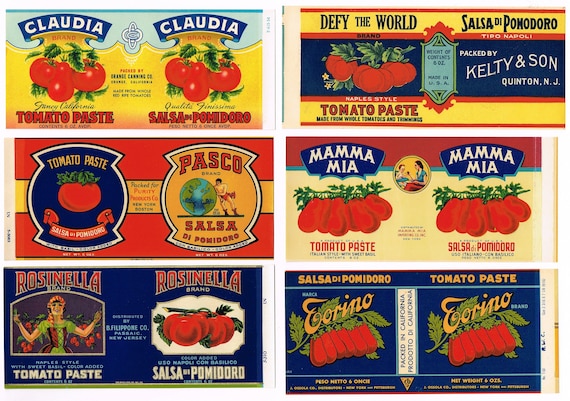The image is a vibrant, old-fashioned selection of six Italian tomato paste labels, each bursting with bright colors and iconic imagery. In the top left corner, "Claudia" tomato paste is featured with bunches of red tomatoes and green leaves against a yellow background. The top right label, "Defy the World" by Kelty and Son from Quinte, New Jersey, showcases red tomatoes and green leaves with a yellow and dark blue backdrop.

The middle row starts with a label from "PASCO," displaying a man leaning against a globe next to red tomatoes and green leaves, with a mix of yellow and red hues. Adjacent to it is the "Mamma Mia" label, which vividly shows a woman feeding a child, surrounded by tomatoes and leaves on a red and yellow background.

In the bottom left corner, "Rosanella Brand" from Passaic, New Jersey, depicts a woman in a green dress with raised hands, set against a deep blue background filled with tomatoes. Lastly, the bottom right corner features "Torino" tomato paste with a white stripe indicating it's packed in California. This label presents long tomatoes with green leaves on a predominantly blue background.

Altogether, these labels present a rustic and colorful feel typical of traditional Italian food packaging, predominantly using red, yellow, and blue colors to attract the eye and evoke a sense of nostalgia and quality.